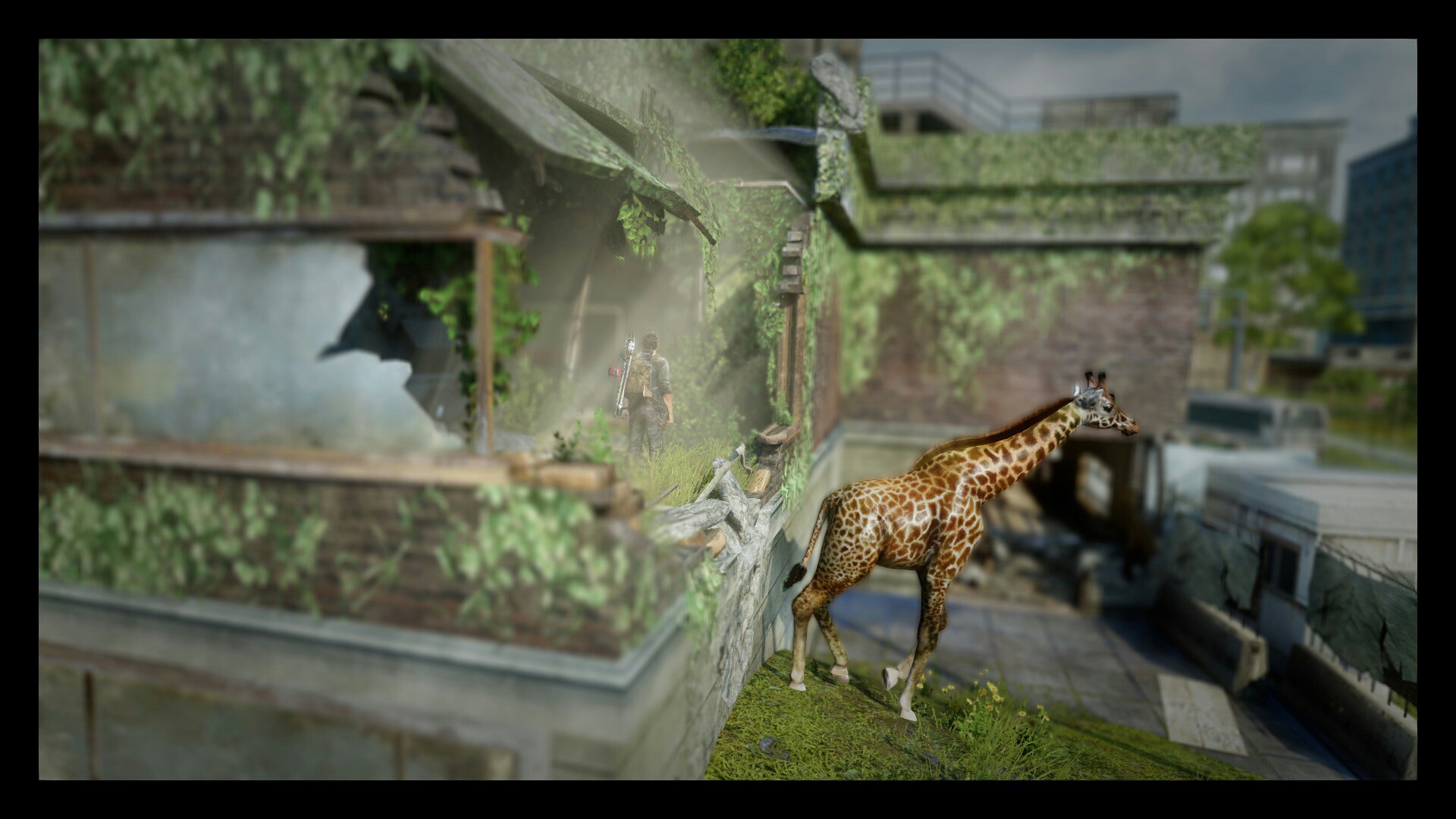This image, which appears to be a highly detailed model, captures a captivating scene of a miniature giraffe walking out of the open door of a large, stone house. The house is in a somewhat ruinous state, missing one entire wall. In the shadows, several tiny figures stand, adding an element of intrigue. The structure, possibly once a greenhouse, features a large window and is filled with lush greenery, including trees and branches. The overall scene is dominated by verdant hues of green, complemented by patches of grass. The giraffe is making its way towards what seems to be a wall or possibly a gate. The sky in the background boasts a grayish-blue tone with an overtone of gray, imbuing the scene with a somber atmosphere. The perspective is taken from the corner of the building, providing a view down the length of the structure towards the opposite end.